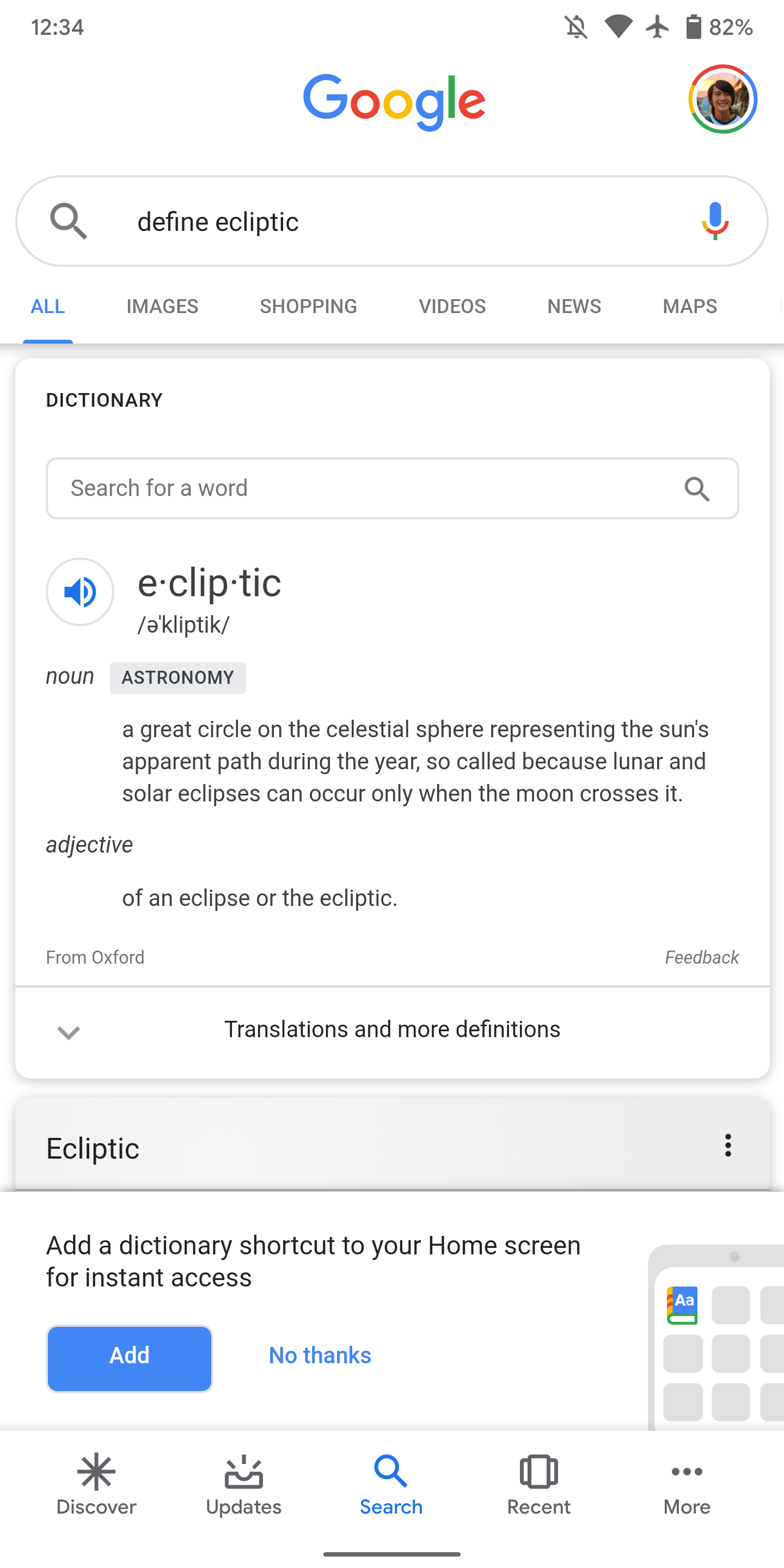The image is a screenshot taken from a cell phone, displaying the time at 12:34 PM on the upper left-hand side of the screen. The phone's status bar shows the Wi-Fi icon, airplane mode icon, and a battery level at 82%. Below the status bar, the word "Google" is center-justified at the top, followed by a search bar containing the query "Define Ecliptic".

Directly beneath the search bar are various navigation tabs: "All," "Images," "Shopping," "Videos," "News," and "Maps." The screen displays the "Dictionary" section where the word "Ecliptic" is defined. The text describes "ecliptic" as a noun in the context of astronomy, explaining it as a gray circle on the celestial sphere representing the sun's apparent path during the year, termed this way because lunar and solar eclipses can only occur when the moon crosses this path. Additionally, it is classified as an adjective related to eclipses or the ecliptic itself.

At the bottom of the screen, the navigation bar features icons labeled "Discover," "Update," "Search," "Recent," and "More."